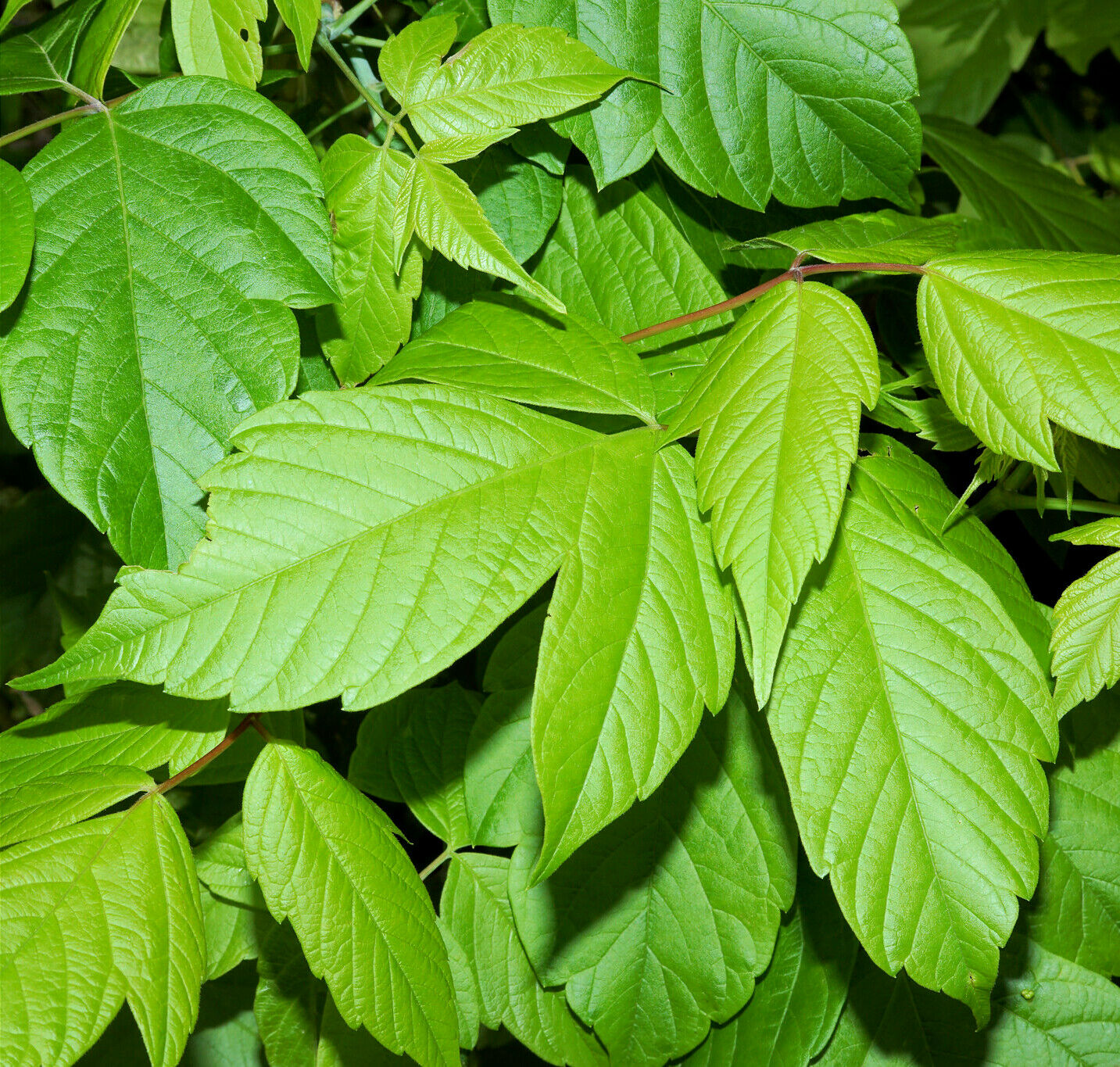This outdoor photograph, bordered between a square and a rectangle, showcases a dense cluster of what appears to be either poison oak or poison ivy. The foliage, piled thickly, includes a variety of green shades ranging from lime to bright. Each leaf, attached to thin stems and discernible tree branches, bears deep lines. Among the multitude of leaves, a few show signs of insect activity, with one distinctly nibbled along the edge, hinting at a beetle's meal. The bright sunlight highlights the front leaves, casting an intricate play of light and shadow as it fades into the darker, thicker background. Aptly captured, this image emphasizes the verdant depth and intricate details of the leafy cluster.